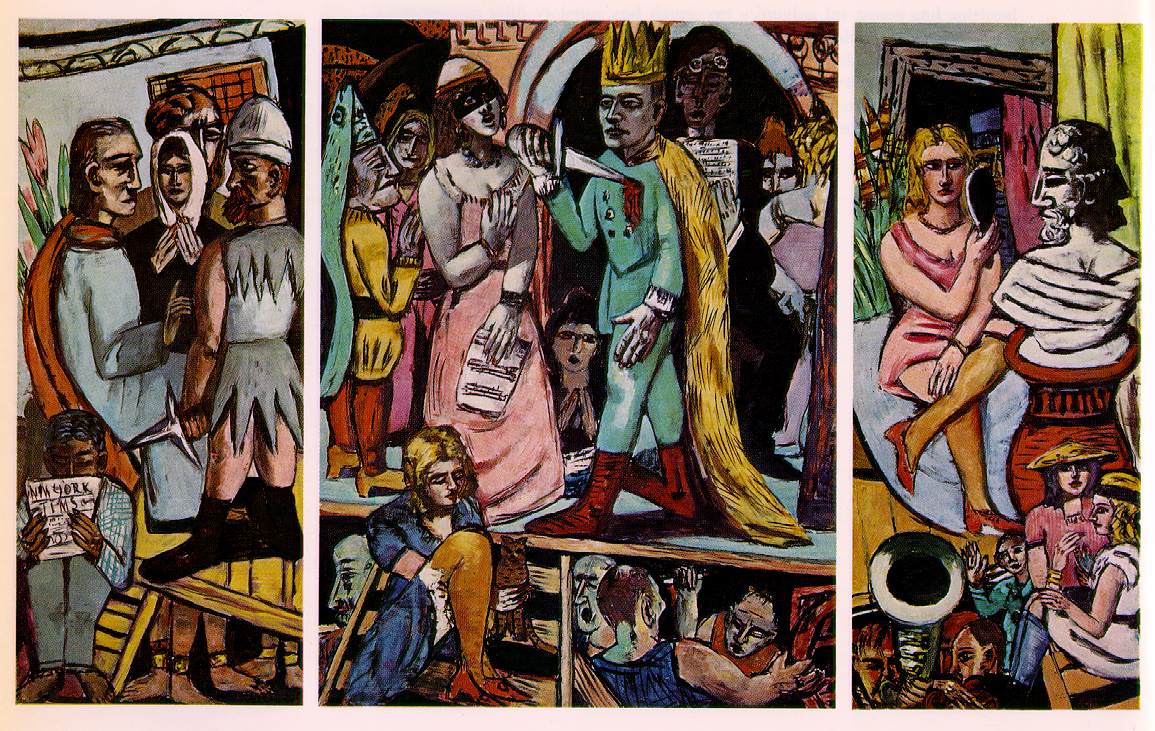This triptych painting, with a blend of medieval and Renaissance styles, showcases three distinct scenes, all interconnected through Shakespearean themes. 

In the first panel, a man in a long blue cloak with a red cape converses with a silver-armored knight standing on a table. A woman in a black robe and pink shawl holds it around her head in the background, while a man in blue and gray clothes sits on the floor reading a paper.

The central and largest panel features a dramatic suicide scene. A king, adorned in green with a golden cape and crown, stands on a platform, stabbing himself in the heart with a dagger. Beside him, a blindfolded woman in a pink dress holds a sheet of paper, her right hand lifted as if addressing the king. Her mouth open suggests she might be singing or speaking. Beneath the stage, a man and a woman sit, gazing up at the scene, while more medievally dressed individuals populate the background.

The right panel depicts someone gazing into a mirror, reflected back is a distinctly Shakespearean "Hamlet's head." A woman in a pink dress with yellow stockings, holding the mirror and adorned with long blonde hair, sits on a bed beside an all-white statue. Below the platform, more figures interact, contributing to the painting’s overall medieval sketch-like yet vivid quality. The muted yet varied color palette includes greens, blues, pinks, golds, tans, grays, and blacks, enhancing the scene's intricate details and artistic depth.